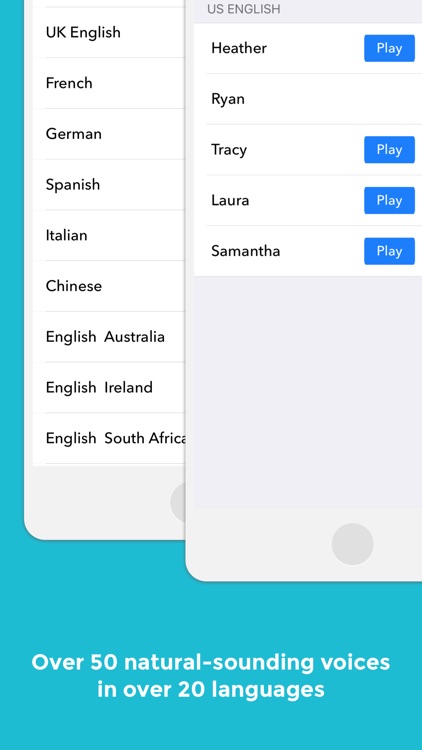This is a detailed and clean caption of the image described:

---

Screenshot from a language learning or speech synthesis platform. The background is a soothing sky blue or Caribbean ocean blue. At the top, text in bold white reads, "Over 50 natural-sounding voices in over 20 languages." Below this, two drop-down menus provide various options for language and voice selection.

The first drop-down menu, positioned on the left, lists multiple languages vertically with thin lines separating each entry. The languages include: UK English, French, German, Spanish, Italian, Chinese, English (Australia), English (Ireland), and English (South Africa).

To the right, the second drop-down menu is set to US English, displaying a list of voices: Heather, Ryan, Tracy, Laura, and Samantha. Each name is accompanied by a blue button with white text that says "Play," allowing users to preview voice samples, except for Ryan, whose option does not have a play button.

The platform appears to offer a wide range of natural-sounding voices, possibly for the purpose of selling these services or integrating them into another system for users.